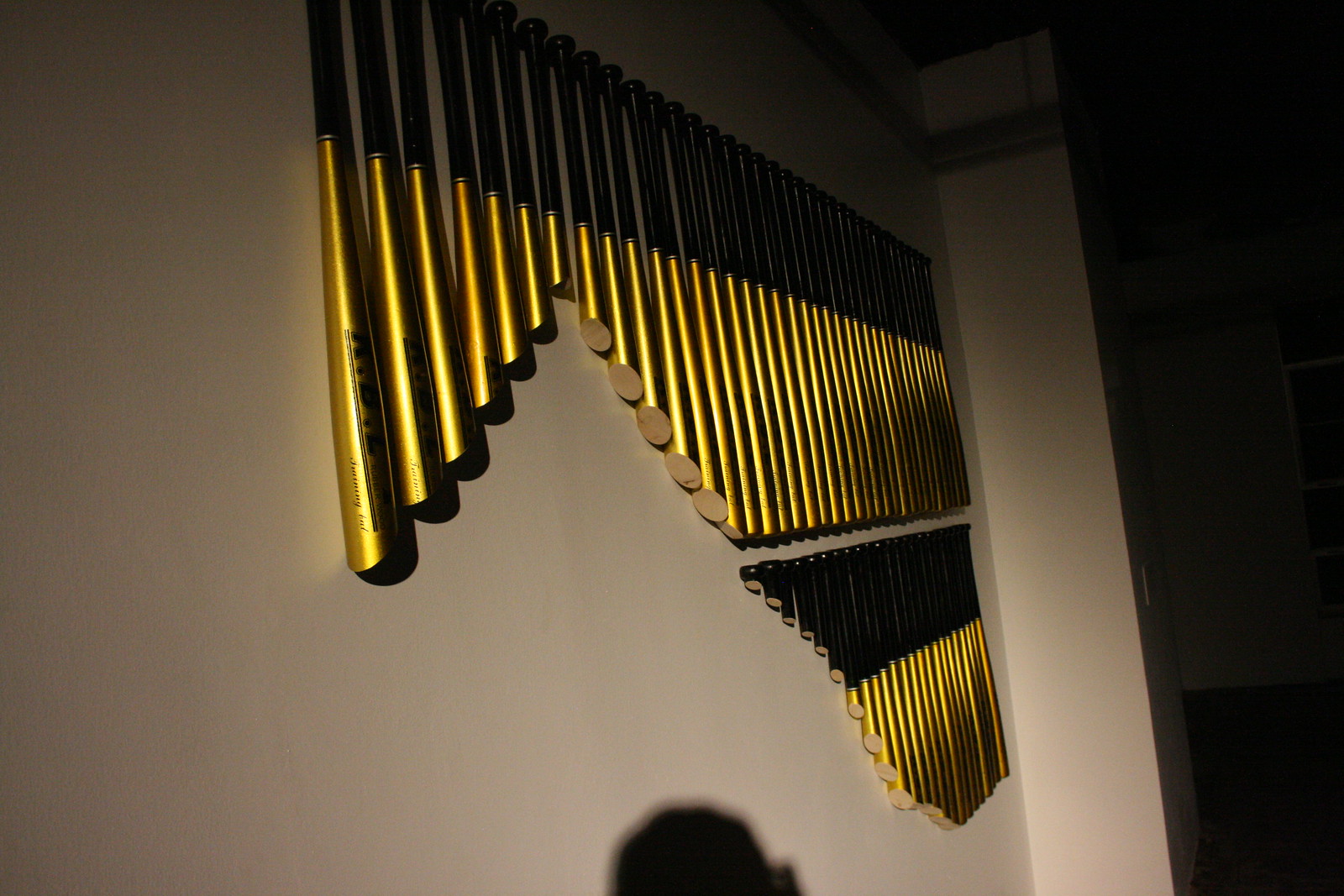This image captures a striking art installation on a plain white wall, featuring a meticulously arranged series of glossy gold baseball bats with black handles. The display comprises two rows, with the upper row housing approximately 50 bats mounted vertically, and the lower row containing around 25, each bat placed directly below the upper bat. The bats form a pattern, where cuts create a triangular space, starting at the left end of the upper row and tapering down to a point slightly left of center. This cutout disrupts the uniform length of the bats, with the long, uncut bats flanking the shorter, triangularly-cut bats. The triangular negative space continues down into the lower row, explaining the fewer bats there. The lighting in the room casts a soft glow on the display, and a shadow, presumably of the person taking the photograph, is visible at the bottom center of the image.